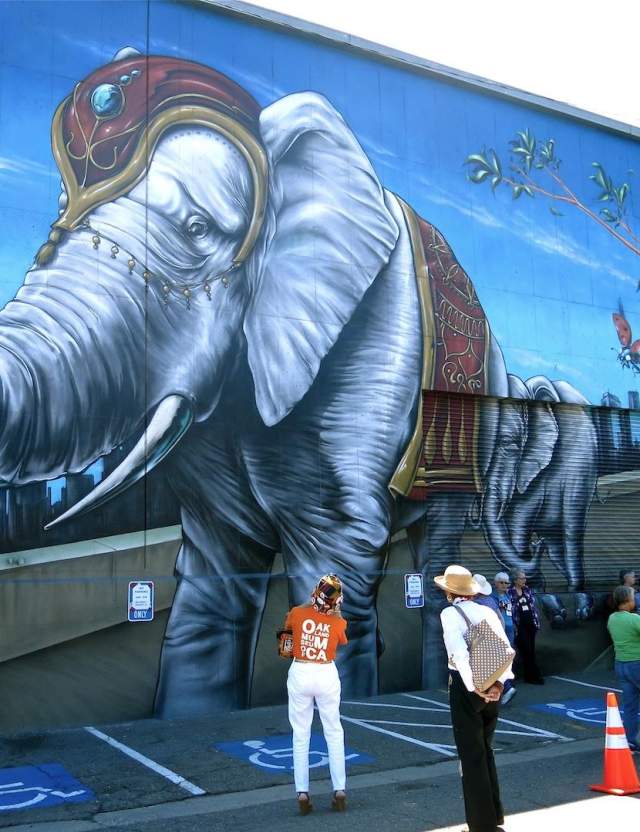In this outdoor photograph, we see a striking mural adorning a large city wall, brilliantly depicting two elephants, likely a mother and her calf. Both elephants are intricately adorned with decorative cloths, featuring muted shades of red, gold, and dark purples, and elaborate headdresses that evoke a regal or ceremonial aesthetic. The sky in the painting is a vivid blue, which complements the blue and gray tones of the elephants themselves. 

In front of the mural, a woman, dressed in an orange t-shirt and white pants, is prominently positioned, appearing to capture a photo of the artwork. Nearby, a man in a straw hat and holding a bag over his shoulder, along with other onlookers, gaze up at the mural, underscoring its appeal as a tourist attraction. The ground, marked with grey hues, features clear signs indicating disabled parking spaces, including the blue and white wheelchair symbols. A safety cone rests on the lower right side of the photograph, adding a touch of vibrant orange to the scene. Despite the presence of a few individuals distracted by other surroundings, the mural captivates the attention of many.